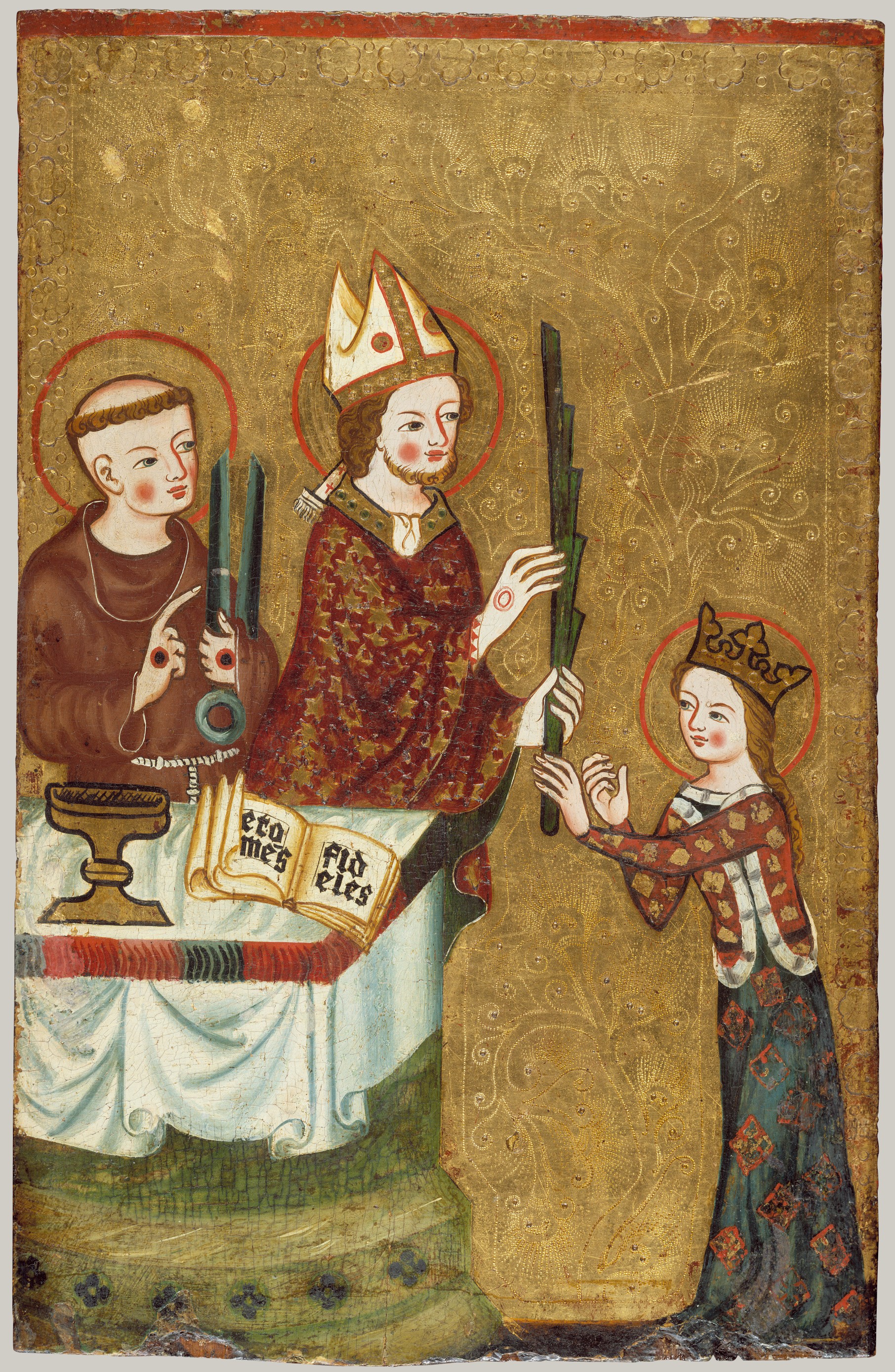The image is a detailed medieval painting likely depicting a religious scene typical of that era. Dominating the foreground is a figure who appears to be a bishop or pope, distinguished by his traditional bishop-style hat adorned with intricate designs, a halo around his head, and a rich, reddish robe featuring star-like patterns along the front. He is holding a green rod or plant, possibly a palm, though its exact nature is unclear. Next to him stands a serene monk with a shaved bald head and halo, dressed in a brown traditional monk's robe. This monk, who exhibits signs of stigmata with holes in his hands, holds two green rods in his left hand and points upwards. In front of them is a table covered with a white cloth, upon which rests a golden chalice and an open book with Latin or gothic script.

Standing to the right of the bishop, from our perspective, is a young girl or woman, possibly a princess, identified by her crown. She has braided long dark hair, and her attire includes a red long-sleeved top and a green skirt with red diamond shapes. She too has a halo around her head. The background of this painting is a radiant gold leaf, intricately engraved with faint, almost delicate shapes of leaves and trees, providing an ethereal, otherworldly ambiance to the scene. The entire composition exudes a sense of veneration and sanctity, capturing the essence of medieval religious art.